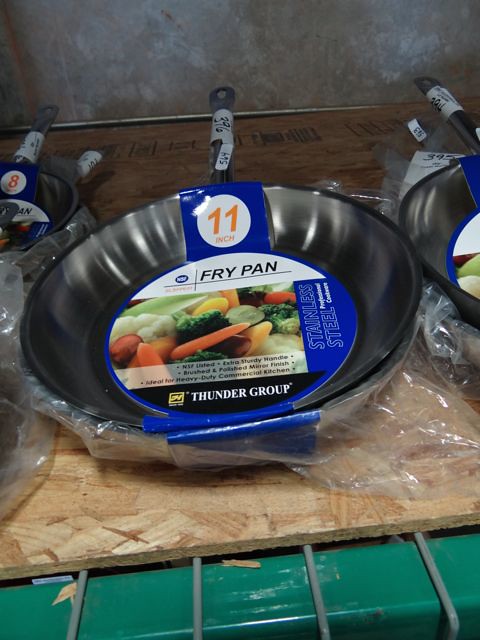This color photograph depicts an indoor setting, appearing to be a kitchen with a green countertop. Central to the image is a piece of pallet wood placed on the counter. Atop the wood is a brand new Thunder Group stainless steel frying pan, still wrapped in plastic with its tags attached, showcasing its 11-inch size. A paper insert within the plastic wrap displays images of vegetables, hinting at its intended use. Surrounding the 11-inch pan are several smaller, also brand new, frying pans. On the left, two 8-inch pans are stacked together, while to the right, there's a 10-inch pan alongside another 8-inch pan. All the frying pans are pristine and unused, reflecting their recent purchase. The scene captures the variety of pan sizes and the newness of the cookware collection.